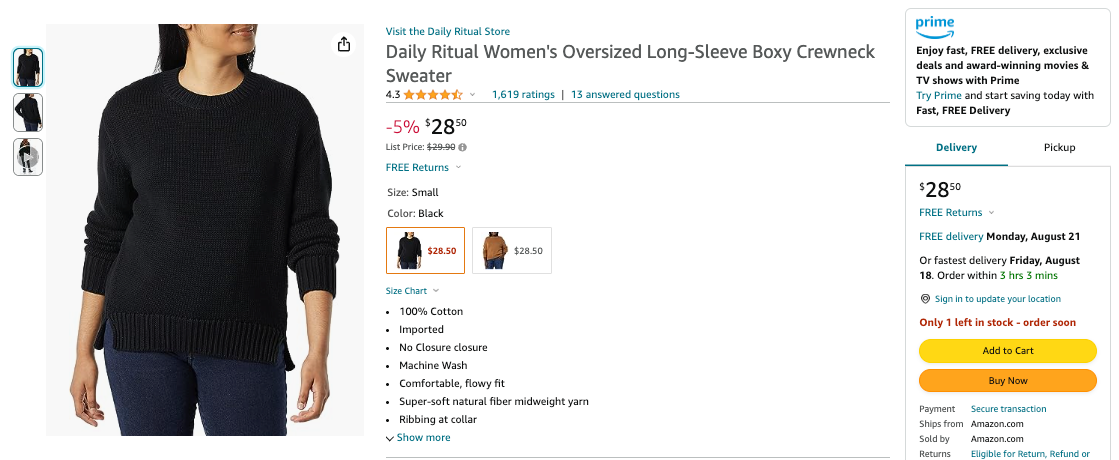The screen capture from the Amazon website showcases the product "Daily Ritual Women's Oversized Long Sleeve Boxy Crew Neck Sweater." The image features a partial view of a person wearing the black version of the sweater, paired with blue jeans. The individual appears to be Caucasian with dark hair, though their face is not fully visible, as the picture cuts off just below the nose, showing only their lips and the bottom part of their ear.

Additionally, a red variant of the sweater is also displayed, allowing potential buyers to select their preferred color before adding the item to their cart. The sweater is currently available at a 5% discount, priced at $28. The product or seller has garnered a rating of approximately 4.3 stars. Customers who choose to purchase the sweater can enjoy free delivery, with an estimated arrival date of Monday, August 23rd, if they opt for the "Add to Cart" or "Buy Now" options.